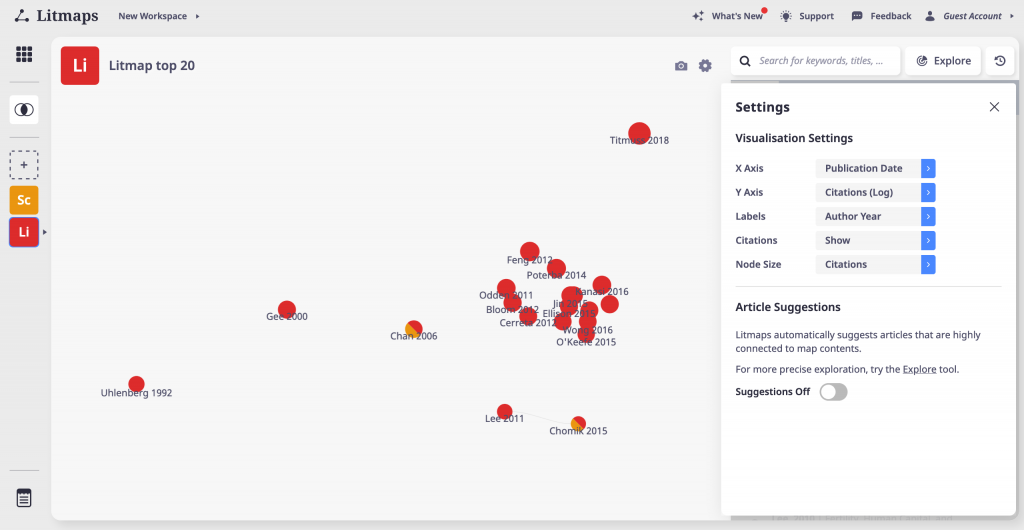In this screenshot, we observe a detailed view of a website interface, specifically a page titled "Lit Maps - New Workspace." In the top left corner, the title "Lit Maps" is written in black text. Top right, the interface displays options in dark gray text: "What's New," "Support," "Feedback," and "Guest Account."

Central to this page is a rectangular map featuring various elements. A square icon labeled "LI" is positioned at the center. To the right of the map, in gray text, it reads "Lit Map Top 20." The map itself is dotted with numerous red circles, representing different areas or names. Notable names include "Li 2011," "G2000," and "Chan 2006," all marked within the map.

On the right side of the page, there is a white box with the heading "Settings" in bold black text. Below this heading, the "Visualization Settings" section is listed with different customization options: "X-Axis," "Y-Axis," "Next Labels," "Citations," and "Node Size." Further down are "Article Suggestions" written in bold dark gray text.

The overall layout appears organized, designed to provide users with extensive mapping and customization tools for navigating literary works or datasets.